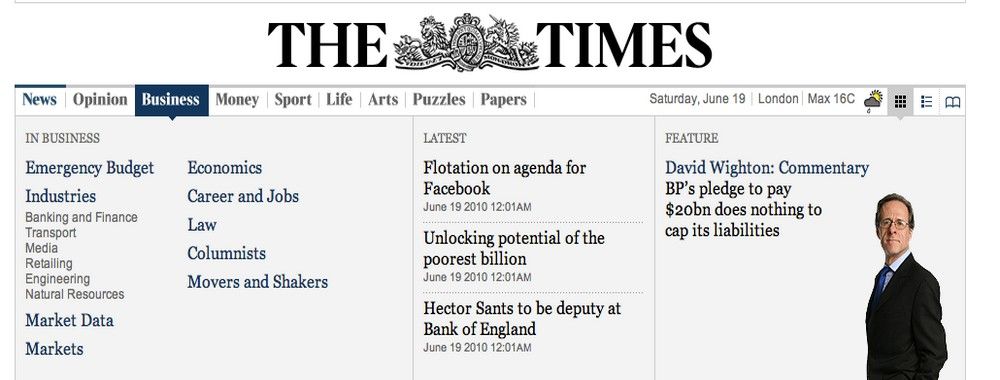The image captures the upper portion of The Times website. Central to the header is the prominent Times logo, elegantly positioned between the two words of the publication's title. Below this header, a horizontal menu bar spans from the left to the right of the screen, listing categories such as News, Opinion, Business, Money, Sport, Life, Arts, Puzzles, and Papers. On the far right, the date of the publication is displayed: Saturday, June 19th, along with the location, London, and the current temperature of 16 degrees Celsius.

The News section appears to be selected, but the focus of the image is on the Business section. Under the "In Business" header on the left side, a variety of links are listed in dark blue text, including "Emergency Budget," "Industries," "Market Data," and "Markets." To the right, additional categories such as "Economics," "Career and Jobs," "Law," "Columnists," and "Movers and Shakers" are presented.

Further to the right, under smaller subheadings, several articles are highlighted: "Latest Flotation and Agenda for Facebook," "Unlocking Potential of the Poorest Billions," and "Hector Sands to be Deputy at Bank of England." Additionally, there is a feature by David Whiten discussing BP's pledge to pay £20 billion.